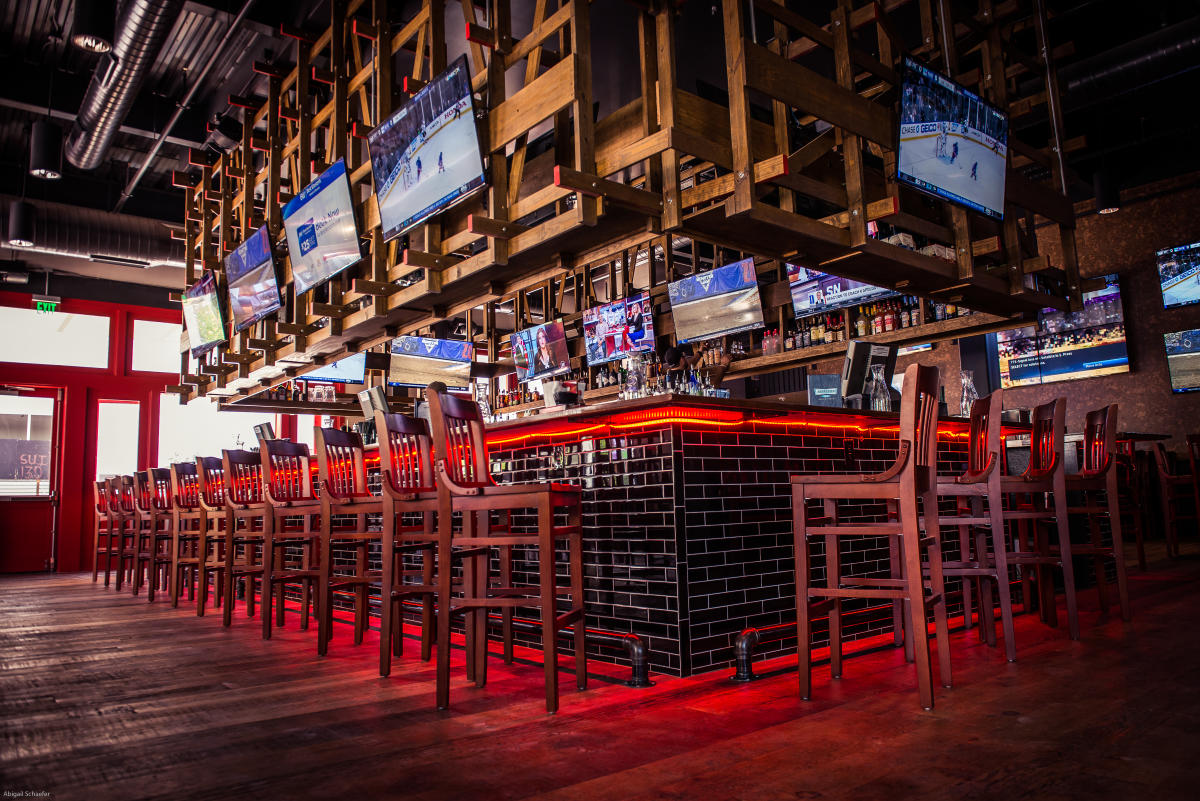The photograph captures the interior of a sports bar with an inviting yet industrial atmosphere. At the center, the focal point is the bar itself, finished with black subway tiles and white grout, accentuated by vibrant orange LED strip lights under the countertop that glow onto the wooden floor. The bar forms a corner, extending both to the left and right, with clusters of tall, brown wooden bar stools positioned diagonally along its length. Above the bar and the rows of assorted liquor bottles, multiple rectangular TV screens dominate the scene, some showing a hockey game and others various broadcasts, suggesting an active sports bar setting. The ceiling features exposed venting, enhancing the industrial vibe, while the upper supports for the screens have a pallet-style design. The scene extends towards the left, revealing the red-trimmed front door and windows, suggesting a glimpse of the exterior concealed by the reflective glass. Despite its ready-for-business setup, the bar stands empty, possibly awaiting patrons for the next opening.